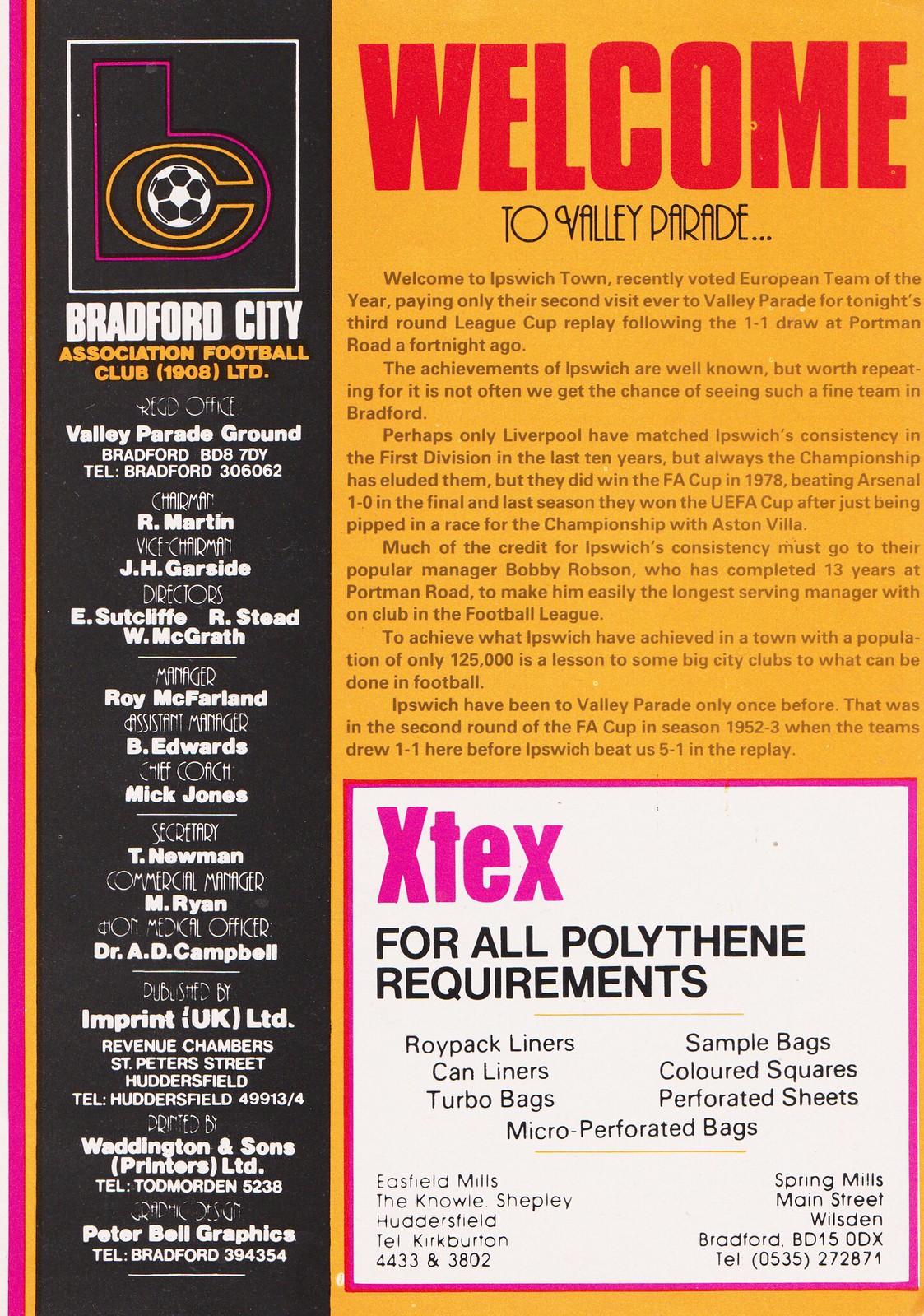The image is a detailed scan of a magazine article. On the left side, a vertical black bar features predominantly white text with a yellow “C” inside a pink “B” emblem containing a black and white soccer ball. Below the emblem, white text reads "Bradford City" and yellow text states "Association Football Club 1908 LTD." Further down, in white text, lists several officials including Chairman R. Martin, Vice Chairman J.H. Garside, and others such as Manager Roy McFarland and Medical Officer Dr. A.D. Campbell.

Adjacent to the black bar, the right side of the page has a yellow background with a prominent red heading "Welcome" followed by smaller black text "to Valley Parade..." The article begins by welcoming Ipswich Town, recently honored as European Town of the Year, as they visit Valley Parade for a third round League Cup replay. It narrates Ipswich's achievements, such as winning the FA Cup in 1978 and the UEFA Cup the previous season, under the management of Bobby Robson. It also recounts their last match with Bradford City during the FA Cup second round of the 1952-53 season.

Towards the bottom right, a white square bordered in pink contains the brand name "XTEXT" in purple font, and black text providing details of their polyethylene products, including various types of liners and bags. The contact information lists Eastwood Mills, Huddersfield, and Spring Mills, Wilson Bradford, along with their respective telephone numbers.